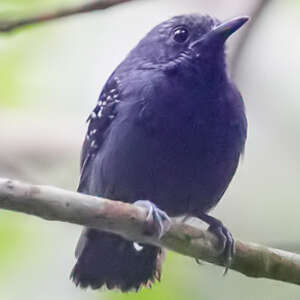In this detailed image, we see a small black bird standing on a branch. The bird features a short, slender black beak and beady black eyes, giving it a contemplative look. Its feathers are predominantly black with delicate white speckles adorning its wings, adding a subtle contrast. The bird's appearance is further characterized by its somewhat puffed-out chest and firmly gripping talons, which are long and sharp to keep it steady on the branch. The branch itself is light-colored with streaks of darker brown, resembling birch wood. In the blurred background, muted tones of light green, white, and gray suggest a wooded area with indistinct tree branches overhead. The overall scene captures a moment of quiet reflection in this bird's natural habitat.